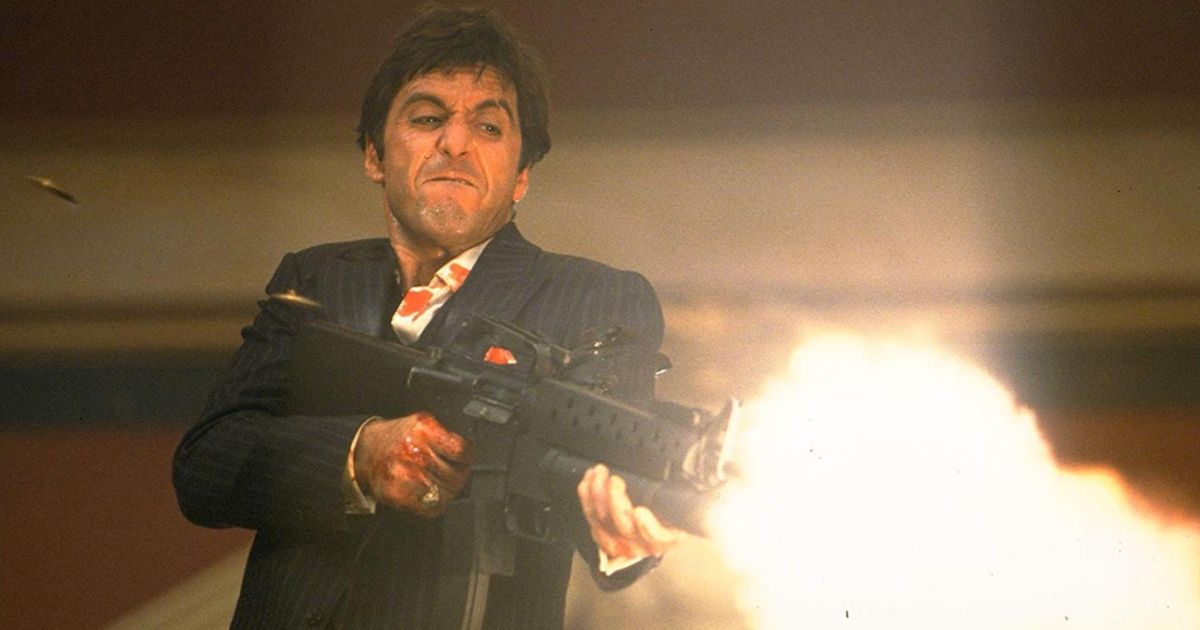This image is a detailed still from the iconic movie *Scarface*, featuring Al Pacino as the main character, Tony Montana. Tony is wielding a high-caliber machine gun, with a fierce muzzle flash illuminating the scene. He is dressed in a dark blue pinstripe suit over a white undershirt, which is stained with blood. Both his hands are bloodied, gripping the gun tightly as he fires, with spent bullets visible in the upper left corner. Tony's face is contorted in a grimace, his brow furrowed and his eyes intense, biting his bottom lip in concentration. He's exerting significant effort, evident from the sweat and strain on his scrunched-up face. He is facing toward the bottom right corner of the frame. The blurred, nondescript background features horizontal stripes with a lighter top half, dark bands, and a tan lower section, suggesting some kind of architectural setting but remaining out of focus to keep attention on the dramatic action in the foreground.